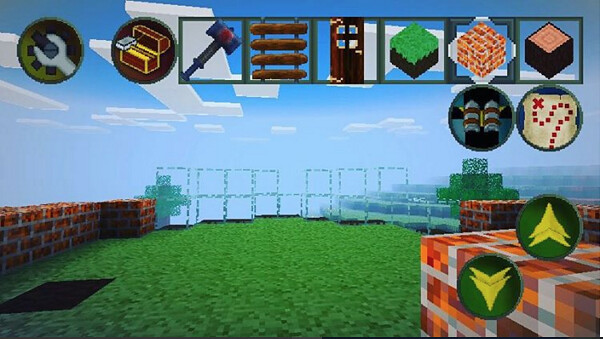This image is a screenshot from a vintage video game, showcasing the simplistic graphical style characteristic of early digital entertainment. The screen layout includes a series of avatar-type buttons and indicators on the sides. At the bottom, there's a green turf, likely representing the ground, adjacent to a reddish brick wall on the left side. In the background, there are open windows and shooting targets, all depicted with basic, low-resolution graphics.

The top of the screen features various avatar symbols and icons such as a wrench, a chest, a hammer, stacked bars, a door, a square, a block, bricks, and several insignias. On the right, there are up and down arrows, a checkered box, and subtle depictions of clouds and sky. The overall scene conveys an early combat or shooting practice game, marked by its simple square shapes and limited color palette, quintessential elements of early video game design.